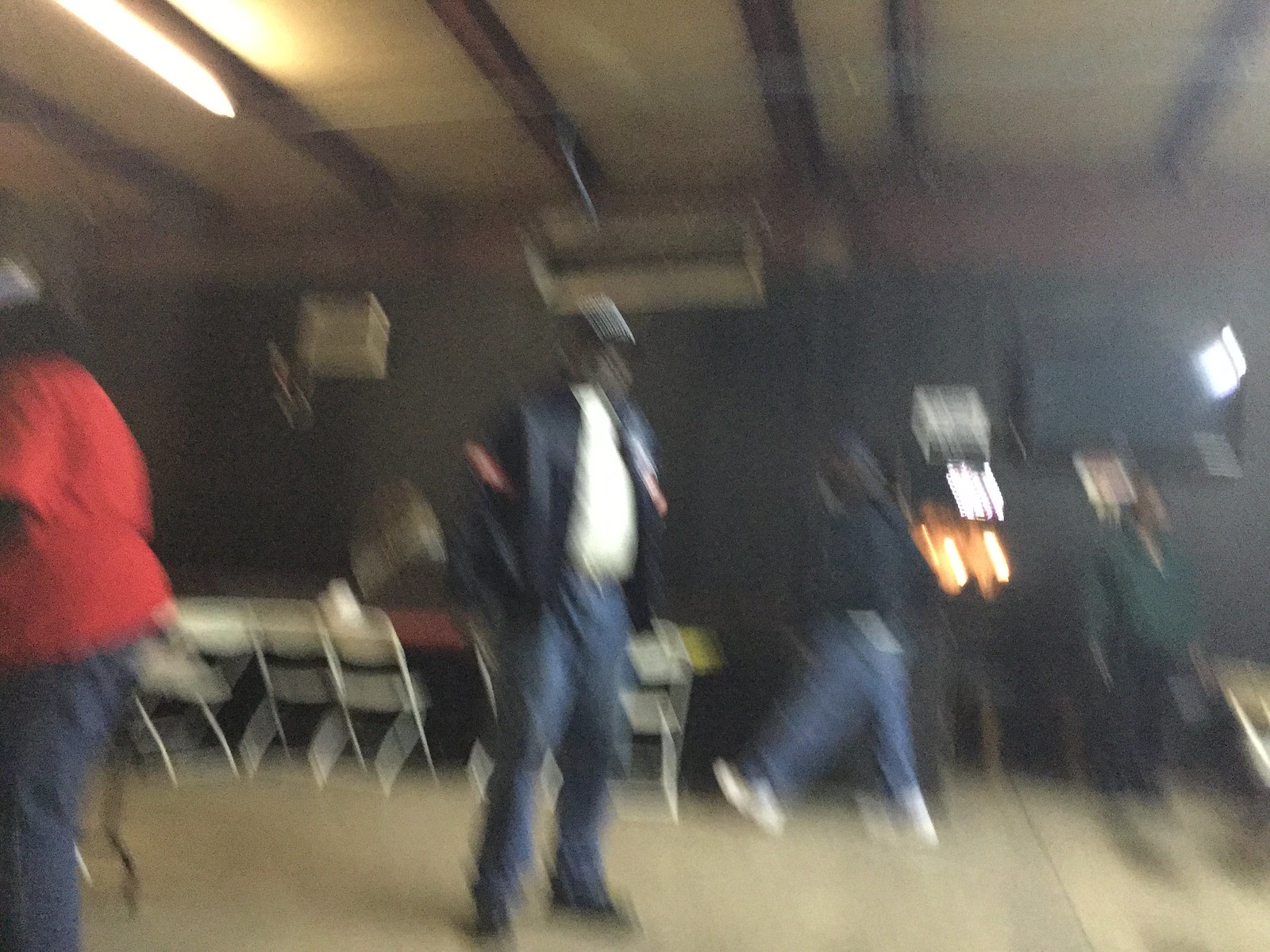In this blurry photograph, a group of people are inside a room with black walls and a light-colored ceiling featuring dark wooden beams. A single fluorescent light hangs from the ceiling, casting a soft glow below. The floor appears to be a light-colored laminate, giving the room a modern feel. 

In the background, there is a long, dark-colored table accompanied by several white folding chairs, approximately four or five in number. To the left side of the image, a large, heavyset person is visible, dressed in dark blue jeans and a red t-shirt. This person has short, dark hair.

Moving towards the center of the image, there is a man with a noticeable beer gut, clad in blue jeans and a dark-colored jacket. His face is unclear, but it appears to be black, and he might be wearing a hat. To his right, a person is captured mid-stride, with their back leg extended and their left foot lifted, suggesting movement. They are wearing blue jeans, white shoes, and a dark coat or shirt, with what seems to be a visible black face.

Further to the right, some blurry light streaks are visible, adding to the overall blur of the photograph. Finally, on the far right, another person stands out, dressed in dark pants, a green jacket, and a white shirt underneath. This individual appears to be a light-skinned black person.

This image captures a seemingly casual gathering in a modern room, with its detailed yet indistinct elements painting a vivid scene despite the blurriness.